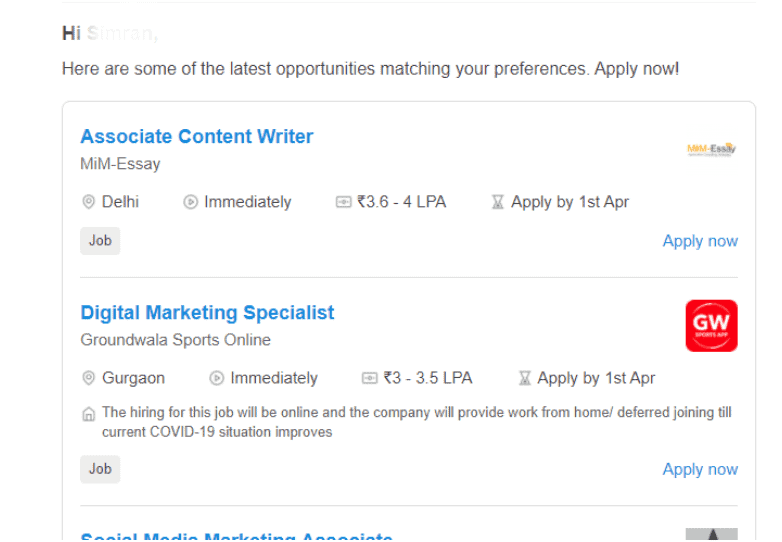**Detailed Caption:**

This image is a cropped screenshot of an email from a job search website. In the top left corner, the email begins with a greeting, “Hi,” followed by a partially edited name that appears to be either "Simon" or "Simran," with remnants of the name still faintly visible. The header text announces, “Here are some of the latest opportunities matching your preferences. Apply now,” in large black font.

Below this header, there is a grey-outlined box containing two fully visible job listings. 

1. The first listing:
   - **Job Title:** Associate Content Writer (in bold blue font)
   - **Company:** MIM-SA (in grey font)
   - **Location:** Delhi
   - **Details:**
     - To the right of the location, there is a coin icon followed by a clock icon.
     - The text "Immediately" follows these icons.
     - Salary Range: 3.6-4 LPA
     - Application Deadline: Apply by 1st April
   - **Buttons:**
     - Bottom left: A grey box with the word "Job" in black font
     - Bottom right: "Apply Now" in bold blue font

2. The second listing:
   - **Job Title:** Digital Marketing Specialist
   - **Company:** Groundwalla Sports Online (in grey font)
   - **Logo:** There is a small square logo of the company in the top right corner of this listing.
   - **Details:**
     - Location, Start Date, and Last Day to Apply are listed.
     - A short job description follows.
   - **Buttons:**
     - Job Listing Button
     - "Apply Now" in bold blue font

The overall layout is organized to provide a clear and concise presentation of the job opportunities, making it easy for recipients to review and act upon the listings.